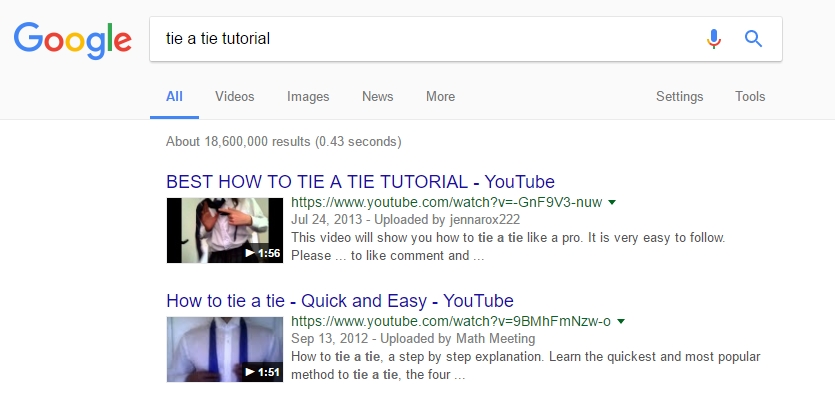The image depicts a Google search results page with a white background. At the very top left, the iconic Google logo is displayed in its characteristic blue, red, yellow, and green colors. To the right of the logo is the search bar containing the query "tie a tie tutorial." Adjacent to the search bar are the microphone and magnifying glass (search) icons. Below the search bar, navigation tabs labeled "All," "Videos," "Images," "News," and "More" are visible, with additional options such as "Settings" and "Tools" on the far right. The search yielded approximately 18,600,000 results in 0.43 seconds. The first two results highlighted are YouTube videos: the top result is titled "Best How to Tie a Tie Tutorial," followed by another video titled "How to Tie a Tie Quick and Easy."